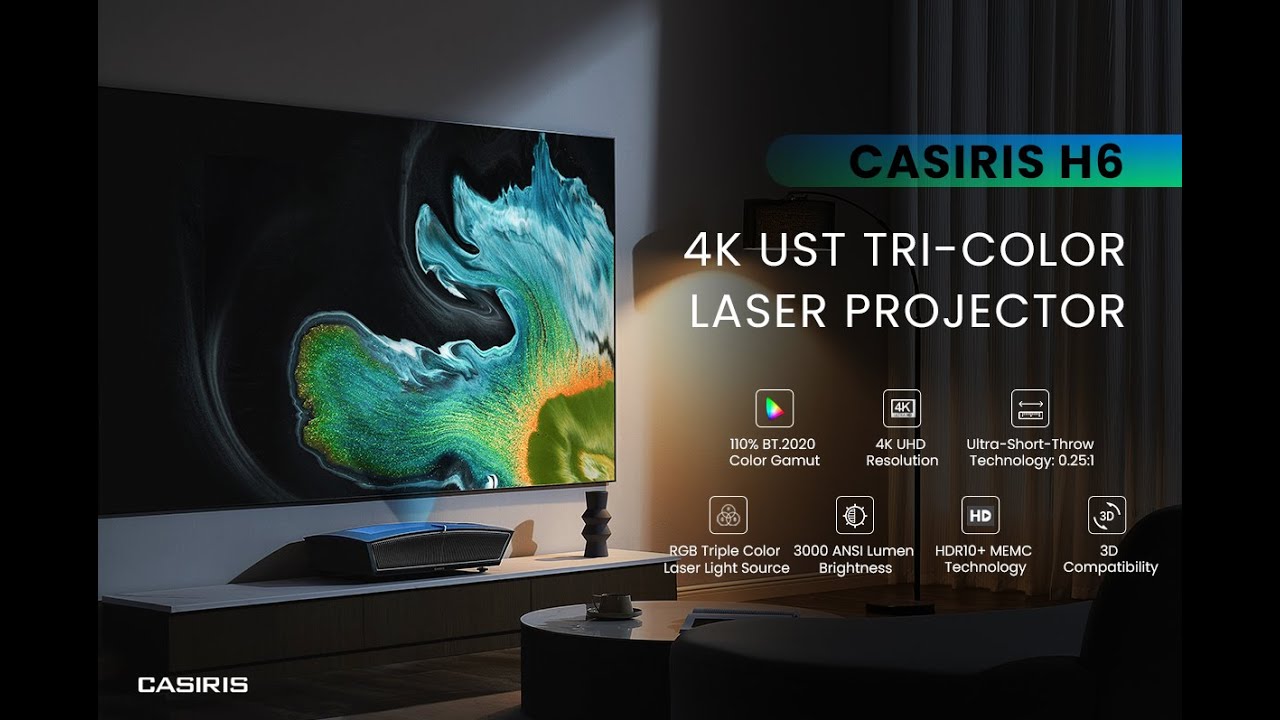The image is an advertisement for the Casiris H6 laser projector. The projector is prominently featured with the brand name "Casiris" (spelled C-A-S-I-R-I-S) visible in white text on a blue and green striped background. The projector offers cutting-edge features including 4K UHD resolution, ultra short throw (UST) technology, and a tricolor laser light source. Additional specifications highlighted are a 110% BT 2020 color gamut, 3D compatibility, HDR technology, and 3000 ANSI lumen brightness. The advertisement showcases a black TV screen above a table, displaying a green ink spill effect to illustrate the vibrant color capabilities. Various icons and text boxes describe these features, emphasizing the projector's advanced technology for an enhanced viewing experience. The ad uses a mix of colors—black, off-white, green, blue, yellow, red, and orange—to draw attention and convey a modern, high-tech atmosphere.